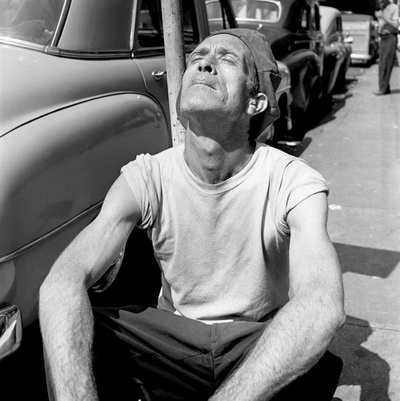In this striking black and white photograph, a man sits directly on a city sidewalk with no visible barrier between him and the pavement. He is positioned beside a row of vintage cars, likely from the 1940s, with about three to four vehicles lined up on the left side of the image. The man, who appears to be around 50 years old, sits cross-legged with his elbows resting on his knees. His head is tilted upwards, eyes closed, as if savoring the warmth of the sunny day.

He is dressed in a white T-shirt with its sleeves rolled up to his shoulders, revealing hair on his arms, and dark work pants. His slightly unshaven face features bushy eyebrows, and his hair is concealed beneath a backward cap. A slight shadow falls behind him, indicating that the sun is shining directly onto his face. Additionally, the faint outline of the car's back passenger side bumper is visible next to him.

In the background, another figure stands on the sidewalk, their head cropped from the frame but their attire—a shirt and pants—still discernible. Overall, the composition captures a moment of seemingly serene contemplation against a nostalgic, mid-20th-century urban backdrop.